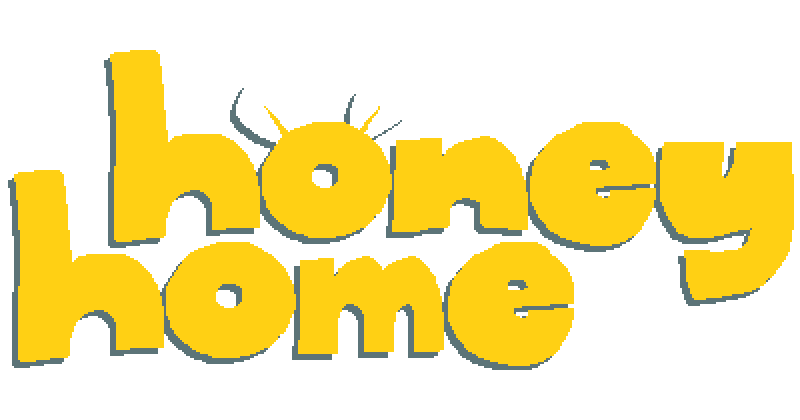The logo for "Honey Home" appears to be a PNG image designed with a charming, handmade aesthetic. Set against a white background, the logo features thick, bold, lowercase letters in a vibrant yellow hue, each accented by a grey drop shadow, giving them a slightly three-dimensional look. The word "honey" is positioned above "home," with "home" indented slightly to the left. Notably, the 'O' in "honey" is adorned with whimsical elements resembling little white wings with yellow accents and a grey drop shadow. The design feels endearingly raw and unpolished, reminiscent of early digital artwork or something hand-drawn in MS Paint. Despite its informal and somewhat clumsy appearance, the logo has an undeniable cute quality that perfectly fits its intended vibe.